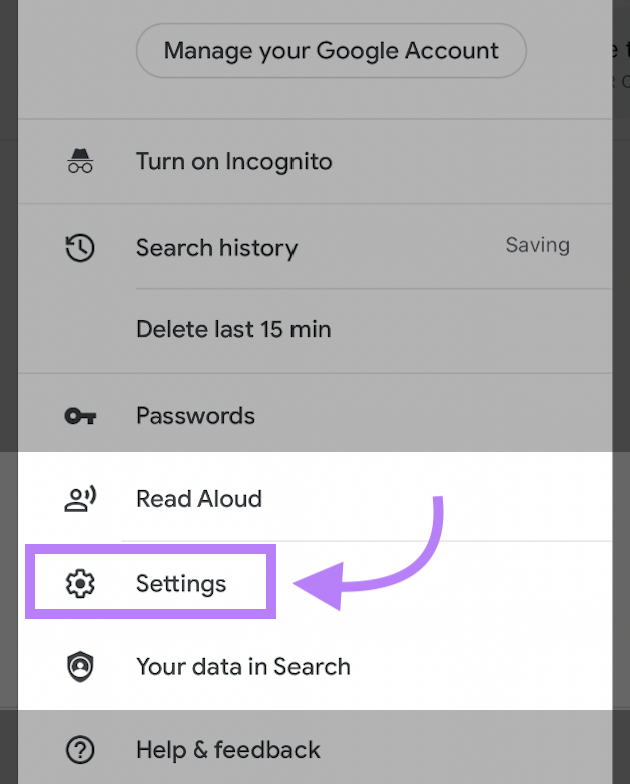**Detailed Caption:**

The image is a screenshot of a website interface featuring a predominantly white background, bordered on the left and right by gray vertical banners. At the top of the page, there is a search bar accompanied by the text "Manage Your Google Account," with each major word beginning with a capital letter: "Manage," "Google," and "Account."

Below this, a series of options are listed, each represented by an icon except for one specific option. The first option is "Turn on Incognito," followed by "Search History," with the word "Saving" capitalized. Next is "Delete Last 15 Min," with "15 Min" written in numeral form (1-5). Following that is "Passwords."

One particular section is highlighted with a white background, prominently showcasing two options: "Read Aloud" and "Settings." The "Settings" option is distinctly marked with a purple rectangle or square, underscored by a purple arrow pointing towards it from the bottom right corner diagonally to the left.

Further down, there is a note that says, "Your search is your data in search," emphasizing user data security and privacy. Finally, at the bottom of the screenshot, within a gray section, are the options "Help" and "Feedback."